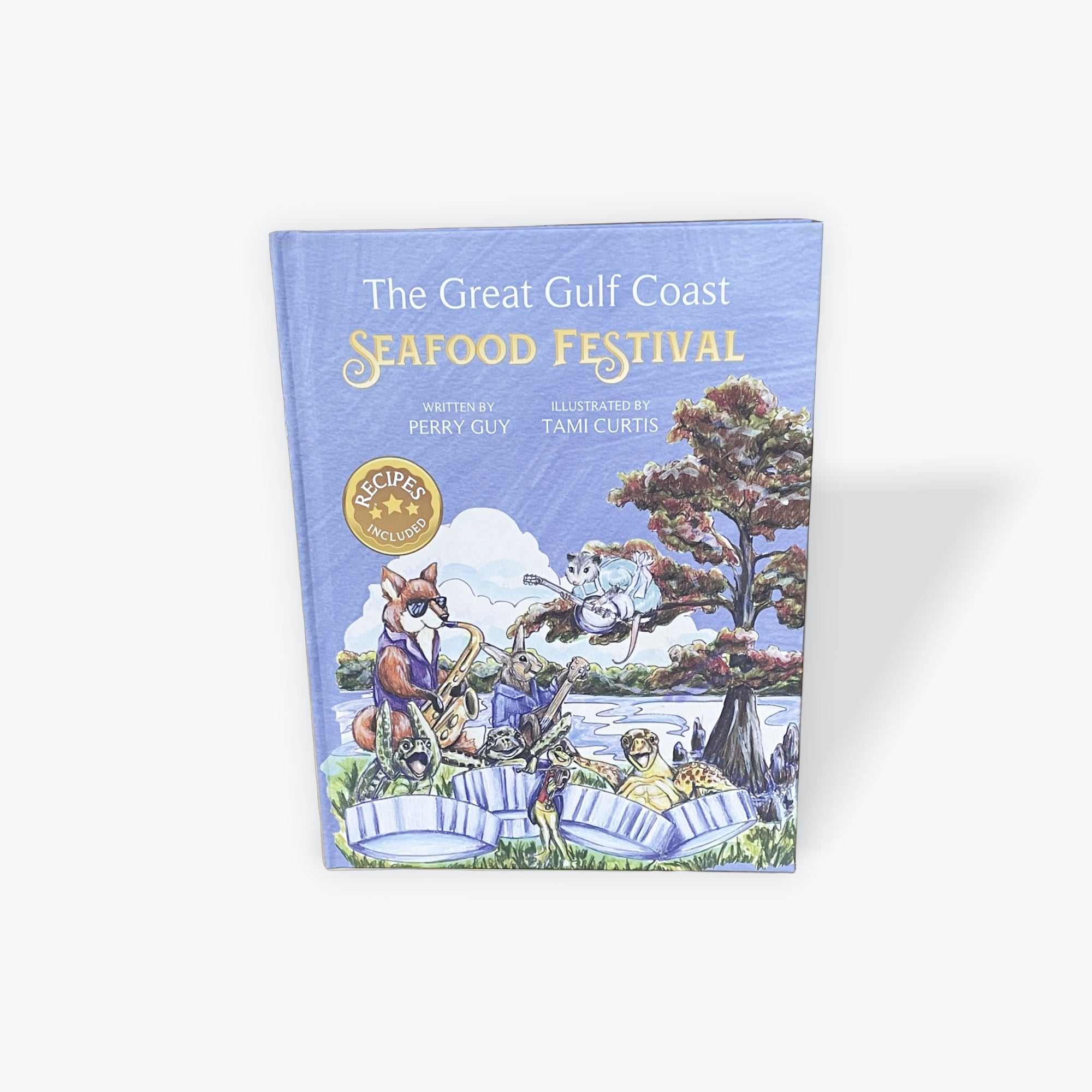The image displays the cover of a book titled "The Great Gulf Coast Seafood Festival," with the title written in prominent white lettering, followed by "Seafood Festival" in gold. Authored by Perry Guy and illustrated by Tammy Curtis, these credits are positioned at the bottom left and right corners, respectively. The cover is rich with vibrant illustrations of animals engaging in a musical performance. Central to the scene, a fox wearing sunglasses plays the saxophone, while a rabbit strums a guitar or a similar stringed instrument beside it. Additionally, a tree adorned with red leaves stands vertically on the right, and within its branches, a beaver-like animal plays another stringed instrument. The backdrop features a cloudy sky and a river with blue and white reflections. Notably, there are four bottle cap-like circles, three of which contain turtles, two of them seemingly excited with arms up, and one possibly posing with arms out, reminiscent of a T-pose. A golden seal above the fox reads "Recipes Included," accompanied by three stars in the center.